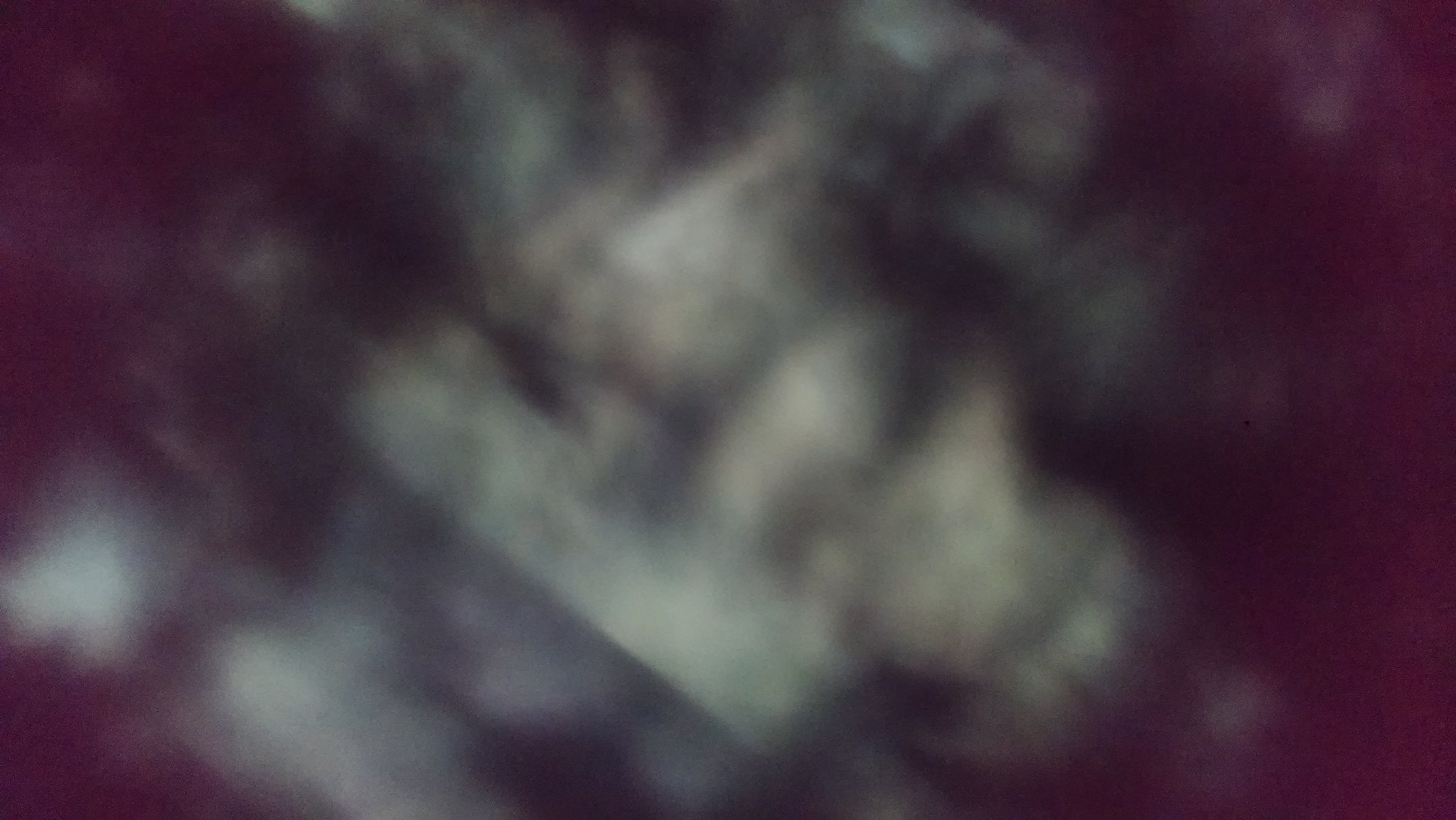The image is reminiscent of an oil painting and is extremely blurry and distorted, making it difficult to discern any clear shapes or objects. Predominantly, it features a mix of deep purple and black tones around the edges, particularly on the left and right sides, which transition into lighter shades of brown, green, and white in the center. This central area appears somewhat paler than the periphery. The ambiguous shapes in the middle suggest a brown figurine holding a plank of wood, though this is not definitive due to the heavy blurring. The image overall is a blend of mottled colors—gray, tan, black, brown—amalgamated in a way that lacks any solid or recognizable forms, resembling a rectangular landscape. The interplay of dark and light hues gives it a cloudy, indistinct quality, with no clearly identifiable subjects or objects.